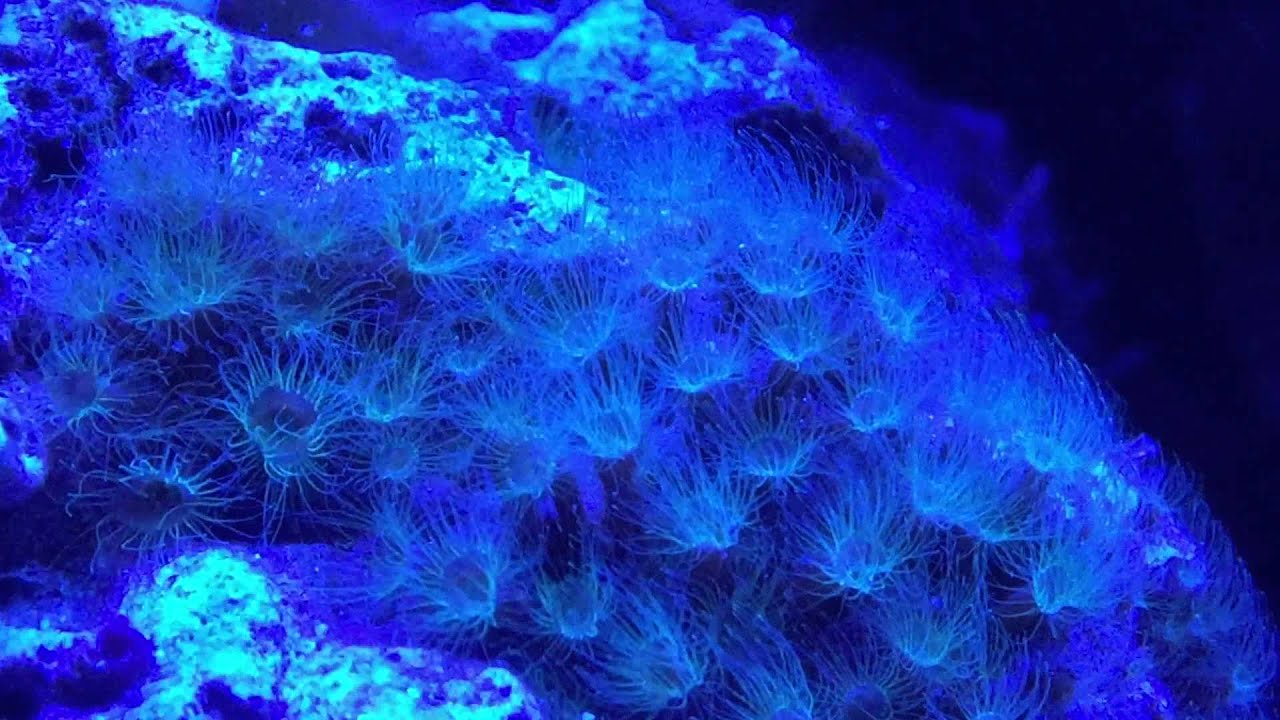This landscape-oriented color photograph depicts a captivating underwater scene centered around a large mass of luminescent jellyfish-like creatures clustered together. Taken in a natural aquatic environment, the image captures dozens of these circular organisms, each adorned with thin, spiny, hair-like appendages extending from their bodies. The creatures exhibit a brilliant blue glow, with shades ranging from lighter to darker blue, creating a mesmerizing contrast against the predominantly dark background. Enhancements of a special blue filter add to the surreal quality of the scene, making the jellyfish appear as if they emit their own light. The upper right corner of the image fades into black, while dappled sunlight discreetly illuminates parts of the cluster, suggesting a light source above the water not visible in the frame. Overall, this detailed and striking photograph showcases a breathtaking glimpse into underwater photographic realism, emphasizing the ethereal beauty of these marine creatures.